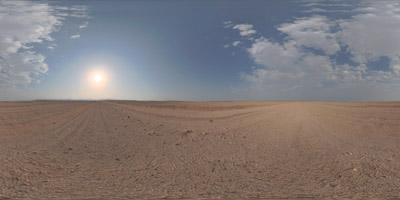The photograph is an intricately stitched panorama, merging two images of a desert landscape taken at different times or from opposite sides of the road. This seamless fusion creates an expansive 360-degree view. On the left, the dirt road stretches forward beneath a blue sky adorned with scattered clouds in the top left corner. The sun is just above the horizon, glowing brightly with a white core surrounded by shades of orange, suggesting it could be either sunrise or sunset. On the right, a second dirt road extends backward, under a cloud-covered sky. The clouds from this side seem to connect seamlessly with those from the left, reinforcing the circular nature of the scene. This detailed panorama captures the tranquility and expansive beauty of a desert at the cusp of day or night.